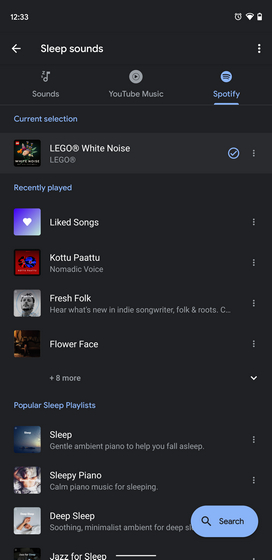A screenshot captures a phone app that integrates multiple music streaming services, displaying the logos of both Spotify and YouTube Music against a dark-themed interface. The app appears to allow users to log in with their credentials from different platforms, consolidating access to various features in one place. The current screen showcases the app’s "sleep sounds" selection, highlighting a playlist titled "Lego White Noise." Additional options under "Recently Played" include tracks like "Katu Patu," "Nomadic Voice," and "Fresh Folk." The section "Popular Sleep Playlists" features various curated lists aimed at promoting sleep, such as "Sleep" with gentle ambient piano music and others like "Sleepy Piano" and "Deep Sleep." Each playlist is designed to help users relax and drift into sleep.